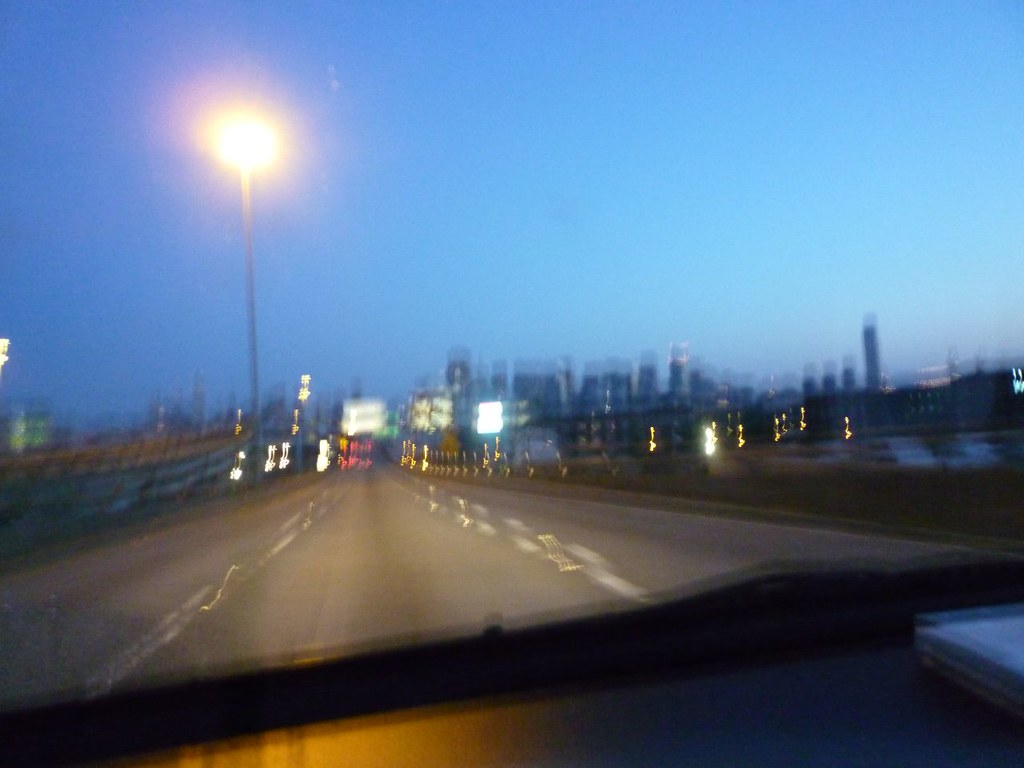Through the car windshield, the scene captures an atmospheric twilight setting, with the dashboard faintly visible. The sky transitions from dark blue to a subtle hint of pink, evoking a serene dusk. The view extends over a three-lane highway, leading in one direction, flanked by road construction on the right and barriers on the left. A single, prominent streetlight stands, casting a yellow glow resembling an orb atop a pole. 

In the background, the silhouette of a sprawling metropolitan city skyline is visible, composed of approximately 25 skyscrapers that stretch across the horizon and blend into the twilight sky. The road ahead appears devoid of other vehicles, with only a few construction signs indicating temporary detours. This tranquil drive through the suburbs edges closer to the bustling cityscape, encapsulating the moment of transition from the outskirts to urban life.